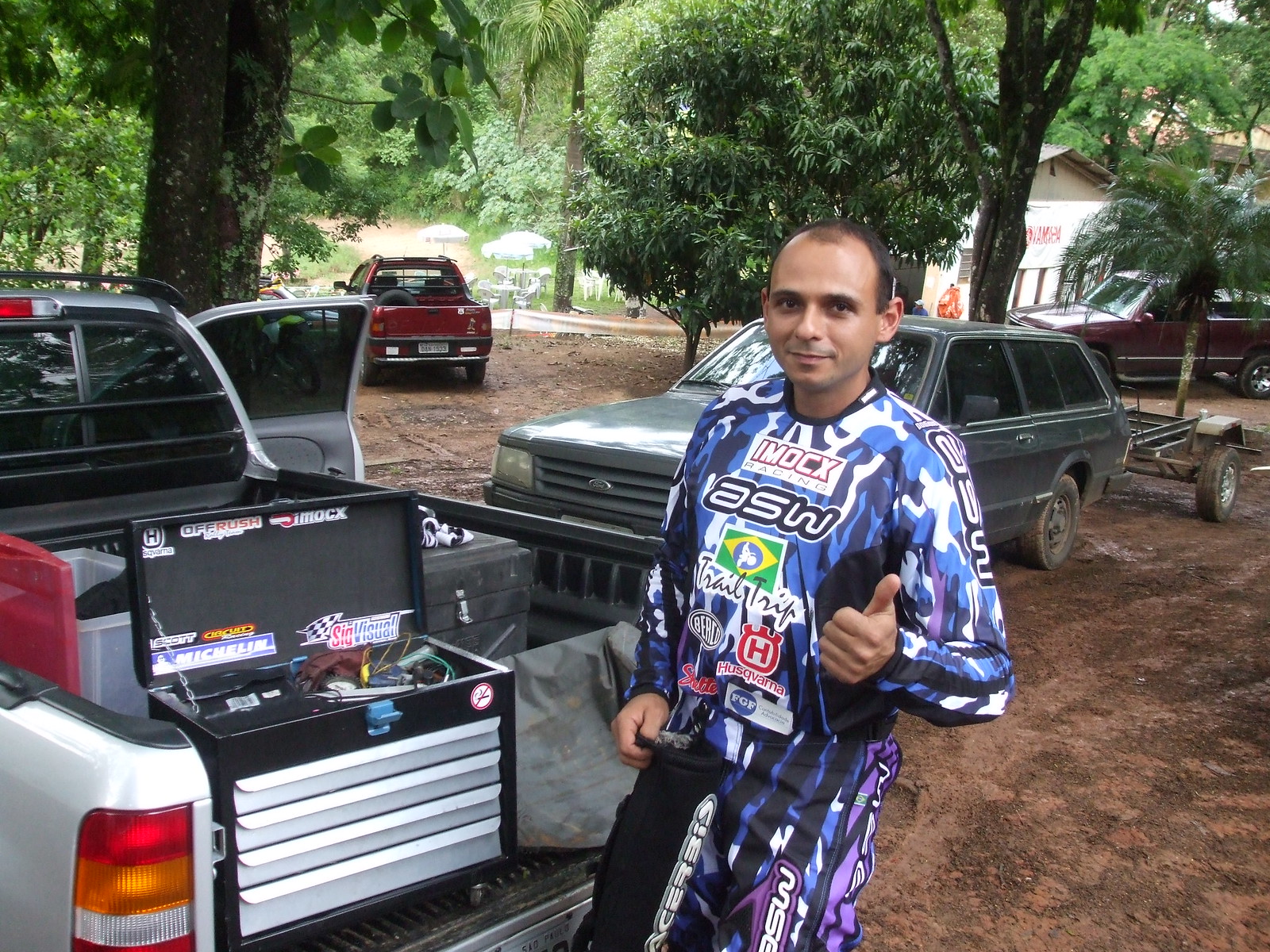In a daylight outdoor setting, a bald white man with short black hair stands in the center of a dirt area under a canopy of green trees, giving a thumbs up to the camera. He is dressed in a distinctive black, purple, and blue camouflage racing suit adorned with various sponsor logos, including "IMOC," "ASW," "Trailer Trip," "HUSQVARNA," "BEACH," "FGF," "MSC," and an illegible "SATDE." To his left, the open bed of a pickup truck, possibly a Ford, reveals a toolbox plastered with decals such as "FRUSH," "IMOCX," a checkered flag with "SIGVISUAL," a "CIRCLUO" sign, a blue and white Michelin sign with "SCOTT," and a no smoking symbol. The background features additional vehicles: a station wagon hitched to a trailer, another pickup truck, and a red pickup truck farther back. The entire scene is framed by greenery and a building with the lettering "JAMEN" on its gabled roof. Umbrellas and tables can be glimpsed near a grassy area adjacent to a dirt road, suggesting a casual gathering or event setting.